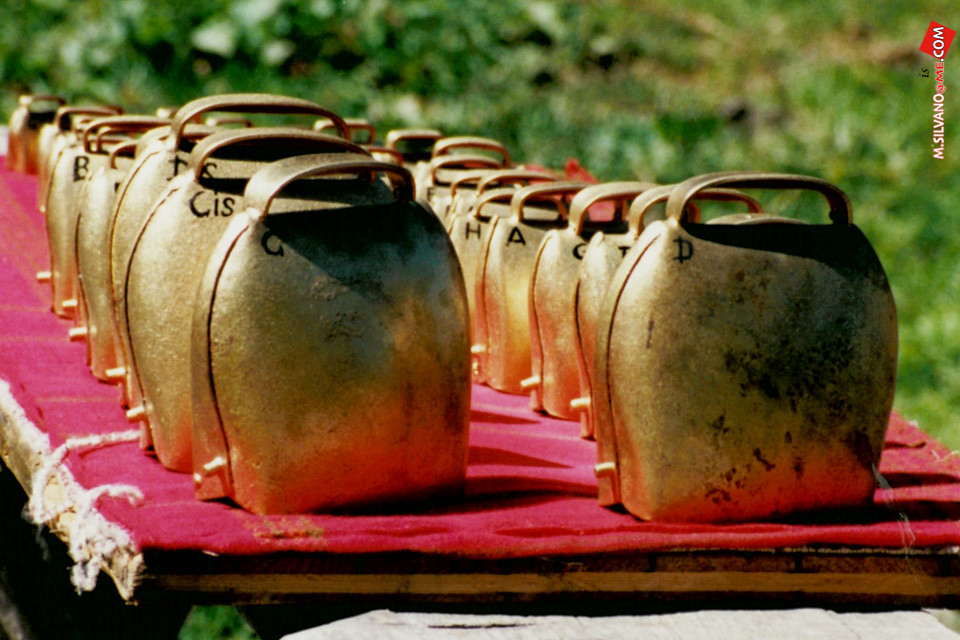In the image, a large wooden picnic table set outdoors is adorned with a thick red cloth covering its entire surface. Resting on the cloth are over 30 large cowbells, which appear to be crafted from slightly rusted metal, possibly brass or bronze. Each cowbell has a handle at the top and features small spouts extending from their left sides. The cowbells are arranged in two orderly rows, with each displaying a unique letter beneath the handle, varying from single letters like A and C to combinations like C-I-S, potentially indicating different pitches or identifications. The setting is lush, with foliage in the background and a grassy area in the foreground, contributing to the rustic and outdoor ambiance of the scene.